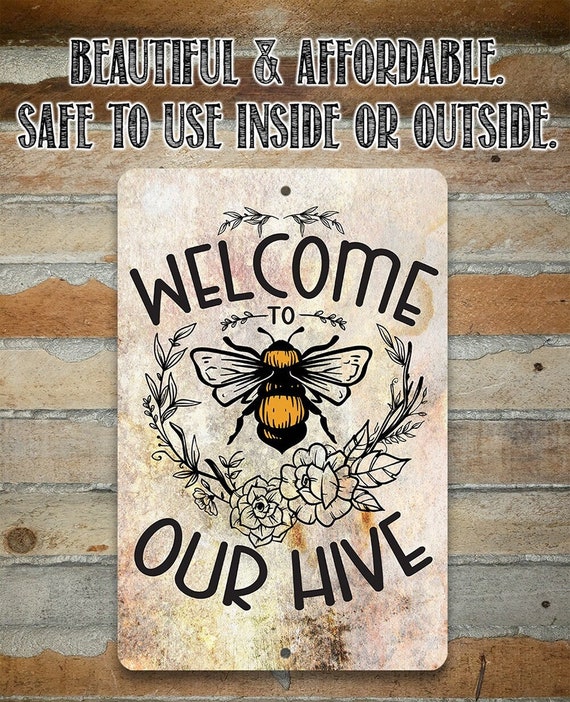The photograph features an old-style house with horizontal light brown wooden slats and gray mortar in between. In the middle of the image, there's a vertical rectangular sign mounted on the wall with visible holes for nailing it. The sign features the black text "Welcome to our hive," with a large drawing of a yellow and black bee with white wings surrounded by a black wreath design, including branches with leaves and two flowers at the bottom. The background of the sign is a mix of beige, pink, and off-white hues. At the top of the image, black and white text reads, "Beautiful and affordable, safe to use inside or outside."